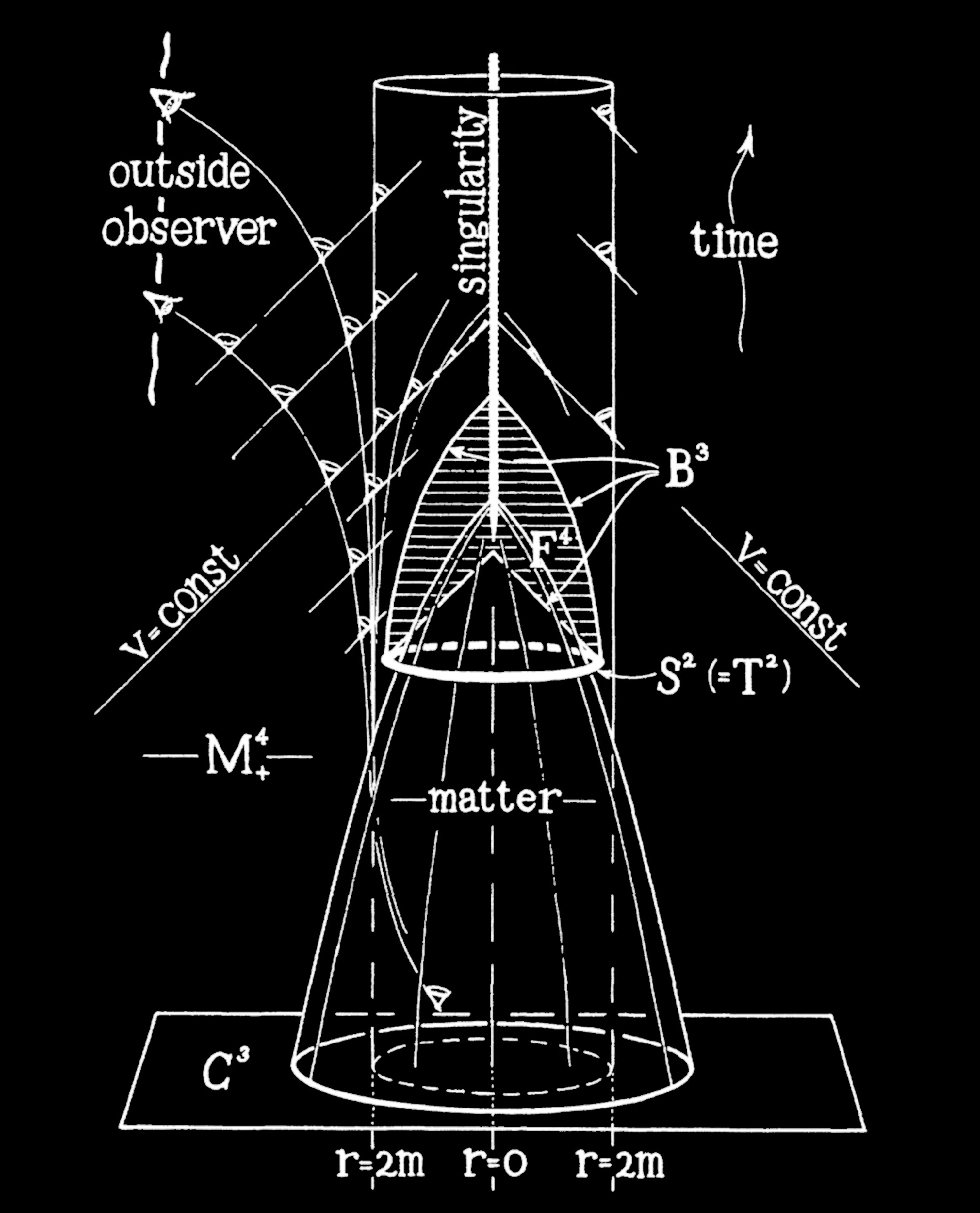This image is a highly detailed scientific diagram set against a black background, with all illustrations and text in white, giving it a blueprint or schematic feel. Central to the diagram is a vertical assembly of geometric shapes: a large inverted cone at the bottom, labeled with "matter" and "M4+", sits atop a rectangle containing two circles. Above this is a smaller cone encircled by a cylinder outline, with the term "B3" at the top.

The diagram features numerous lines and arrows annotated with scientific notations. At the top left, "outside observer" is labeled, with a line leading diagonally downward through the image to "singularity" in the center. The term "time" is annotated on the right, and across various diagonal lines from the periphery to the center, the labels "V = CONST" appear twice. Furthermore, the cone at the base is described by denotations such as "R = 2M", "R = 0", and another "R = 2M". Additionally, within the circumference of the upper cone, mathematical expressions "S² = T²" are noted.

Overall, the diagram appears to illustrate complex physical or engineering principles, possibly explaining the behavior of matter and time as observed from different perspectives.